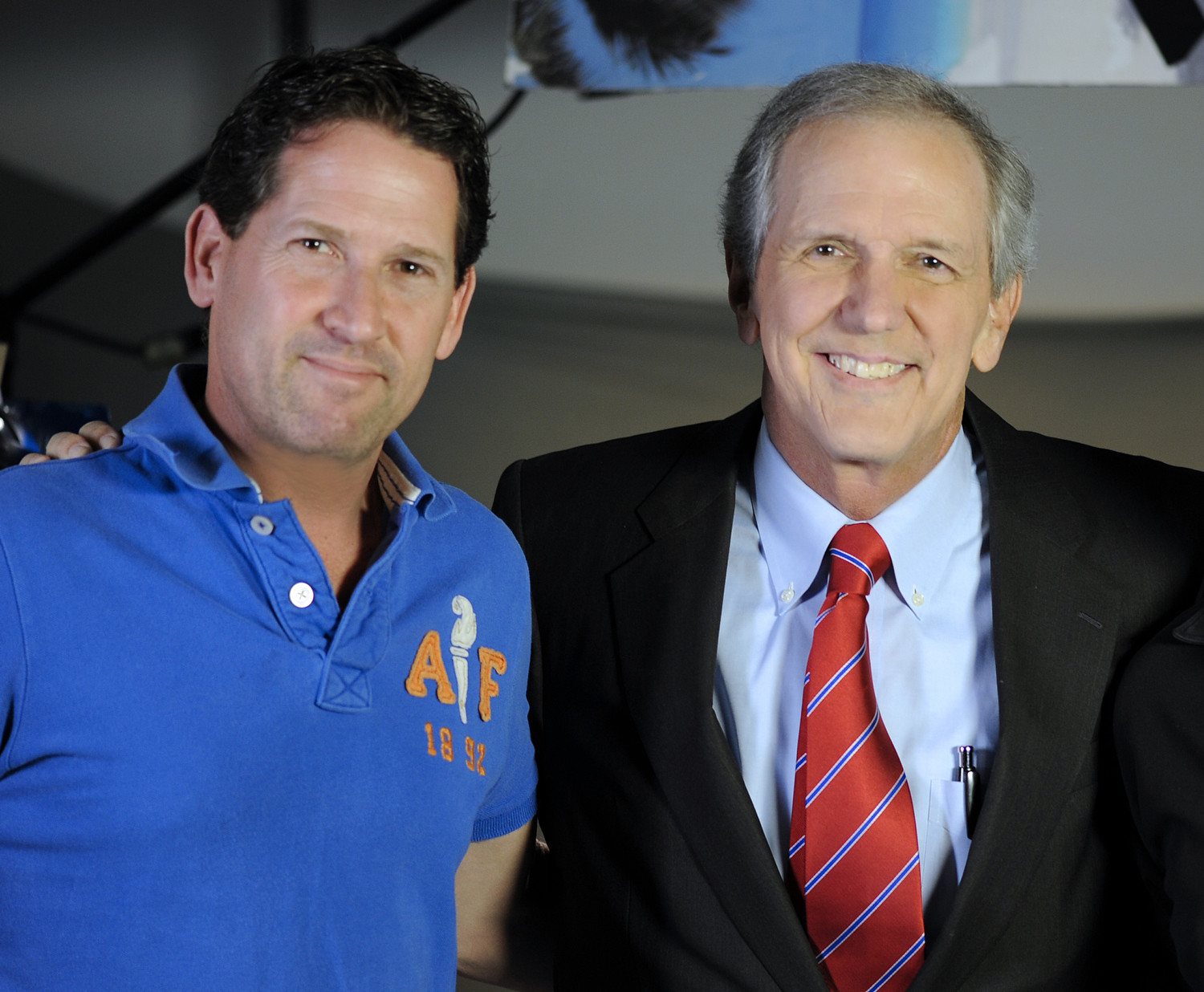The image is a large, square, close-up photograph featuring two men posing for a picture. The man on the left has well-groomed short brown hair, likely styled with gel, and is smiling with his mouth closed. He has brown eyes and is dressed in a blue polo shirt emblazoned with the letters "AF" in orange. Standing to his right is an older man dressed in a business suit. He sports a black suit jacket over a white button-down shirt and a red tie adorned with blue diagonal stripes. The older man has short salt-and-pepper hair, brown eyes, and is smiling broadly, showing his teeth. The background includes a white wall, which might be partially covered by tree branches. Above the older man's head, there appears to be a window through which blue sky and palm branches are visible.